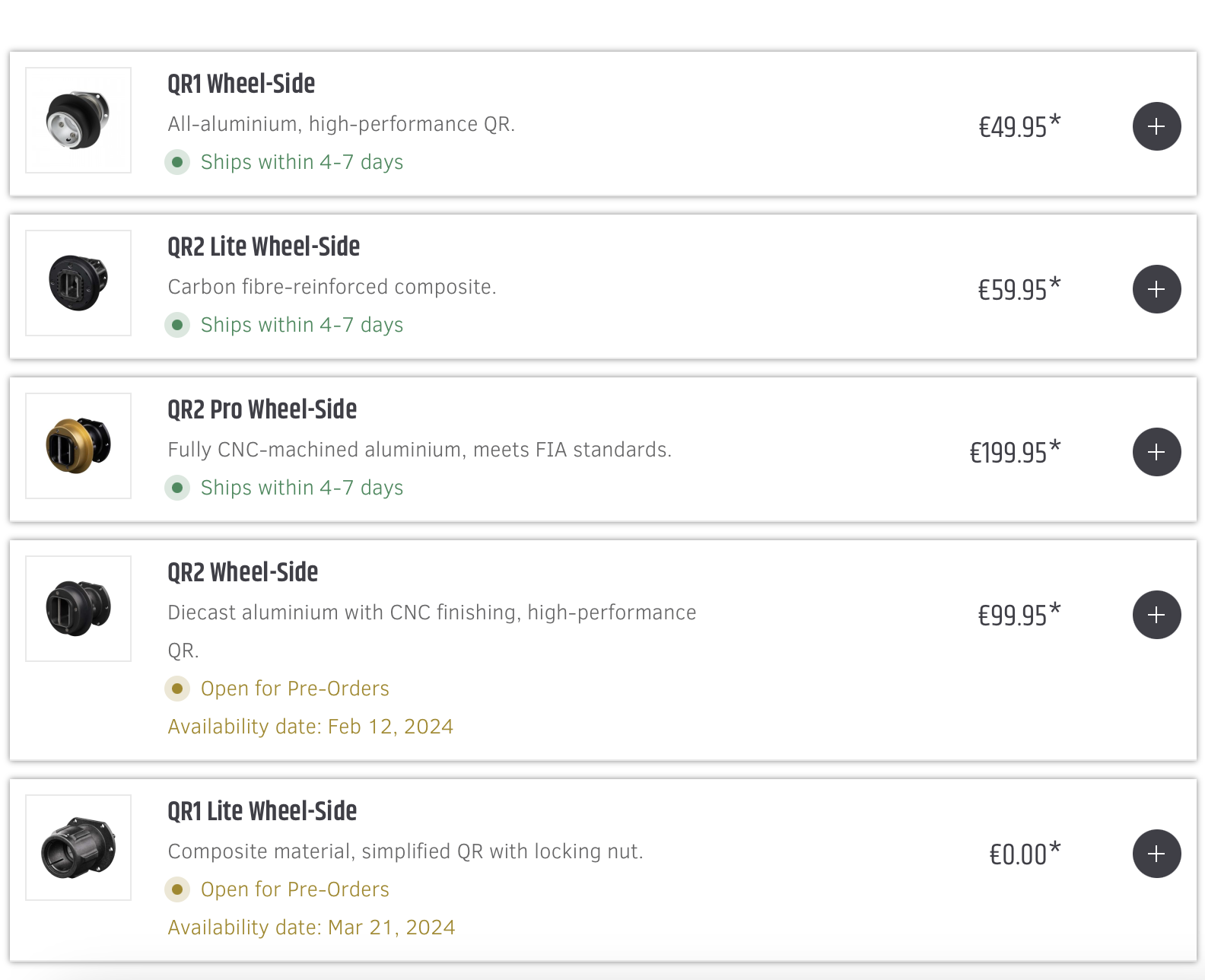Detailed Caption:

This cropped and enlarged image showcases the checkout section of an automotive website, specifically focused on tires. The layout features five distinct white boxes, each displaying a product with comprehensive details. On the left side of each box, there is a photo icon or thumbnail. Adjacent to these images, at the top of each box, are bolded titles describing the product. Directly below the titles, the product details are provided in light grey text. Further down, the estimated shipping time is highlighted in green.

To the right side of each box, the prices are clearly displayed in their own columns. At the far right of each row, there is a black circle with a white plus sign, allowing users to add the respective product to their cart.

The background of the section is a clean white, ensuring that the product information stands out prominently. The first item listed is the "QR1 Wheel Slide All Aluminum High Performance QR," priced at $49.95, with a shipping time of 4-7 business days. Notably, the highest-priced item on the page is the "QR2 Pro Wheel Slide," marked at $199.95. An explanation of this product is provided in a smaller font below its title, detailing its unique features and benefits.